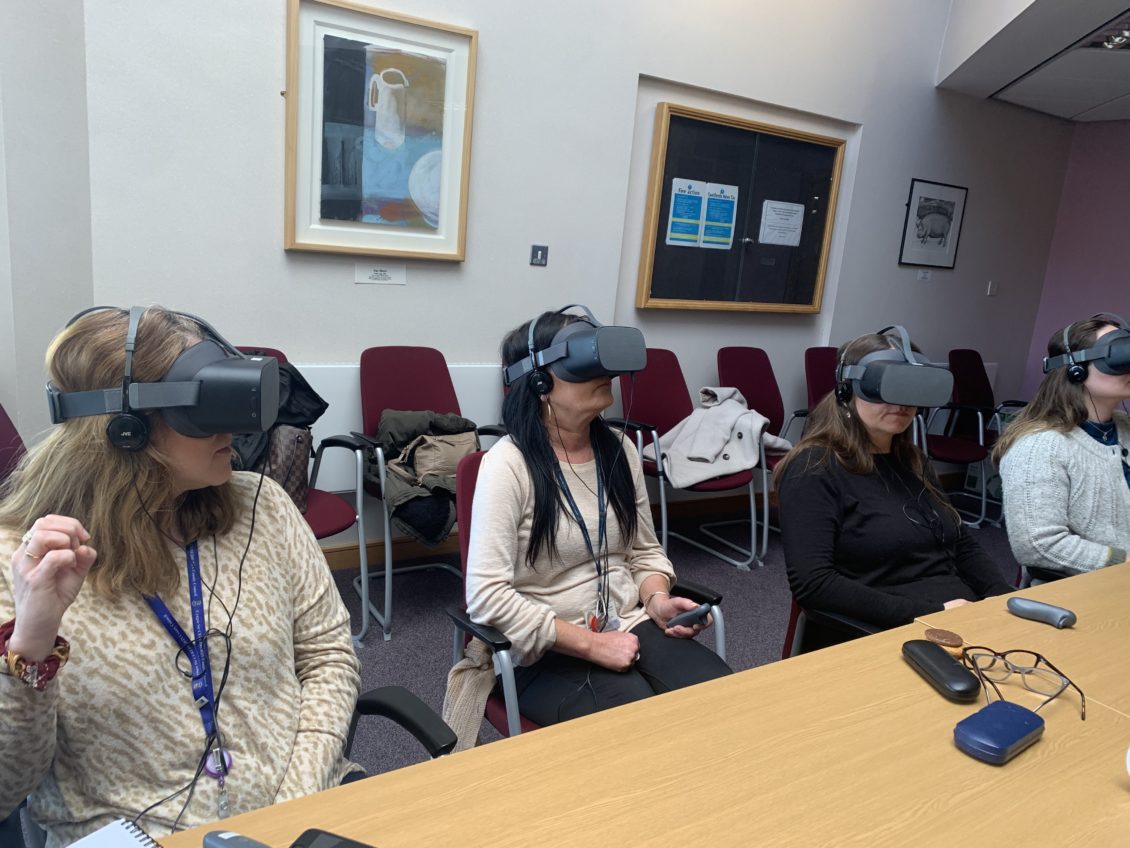In this image, four Caucasian women are engrossed in a virtual reality experience, each wearing black VR headsets that wrap around their heads and cover their eyes, complete with built-in headphones. They are positioned in a setting with a white wall behind them, adorned with a variety of framed items. To the left side of the frame, there is a brown-painted picture frame with a white square and black lettering underneath it. Within this frame is a depiction of a white water pitcher set against a brown background with blue accents below. 

Underneath the picture, the flooring stretches out behind the women, accompanied by a few red chairs, over which some coats are draped. These chairs feature gray legs and black armrests. A brown table sits in front of the women, holding a black and blue glasses case, along with a pair of black and gray-rimmed glasses, presumably set down by the lady at the center.

From right to left, the women are dressed as follows: the first woman wears a white sweater and has dirty brown hair. The second woman, beside her, is dressed in black and also has dirty brown hair. The woman in the center sports a cream-colored top paired with black pants, and she has black hair. The final lady on the far left wears an orange and white top, has dirty brown hair, and a blue tag around her neck. 

Behind these women and to the center of the back wall is a brown frame with a black background, containing two white sheets of paper on the left and one on the right. The sheets on the left feature blue squares with white lettering. Additionally, there is a black-framed picture to the left with a white interior that appears to depict a gray pig. The ceiling above is also white, contributing to the room's bright ambiance. The carpet below is gray, completing the cohesive yet dynamic setting of the scene.